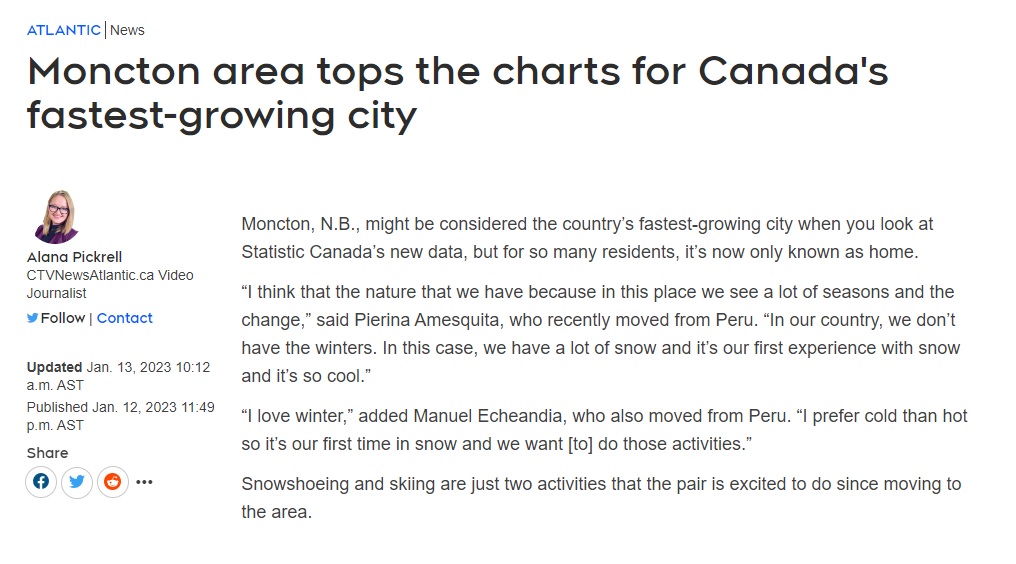This is a detailed caption for the given image:

---

In this landscape-format, color image, a section of an online article from Atlantic News is presented. At the top left corner, the text "ATLANTIC" is prominently displayed in all caps and blue font, separated by a line from the word "NEWS." The article is titled "Moncton Area Tops the Charts for Canada's Fastest Growing City." Written by Alana Pickerel, a video journalist for ctvnewsatlantic.ca, the piece invites readers to follow her on Twitter, or X. The article was updated on January 13, 2023, and originally published on January 12, 2023.

The first paragraph summarizes recent data from Statistics Canada, highlighting Moncton, New Brunswick, as the fastest-growing city in the country. For many residents, however, it’s simply home. The article features quotes from Florina Amasquita, a recent immigrant from Peru, who shares her excitement about experiencing her first winter in Moncton. She says, “I think that the nature that we have, because in this place we see a lot of seasons and the change. In our country we don't have the winters. In this case we have a lot of snow and it's our first experience with snow and it's so cool.”

Another new resident from Peru, Manuel Ekeandia, echoes Florina’s sentiments, stating, “I love winter. I prefer cold than hot. So, it's our first time in snow and we want to do those activities.”

---